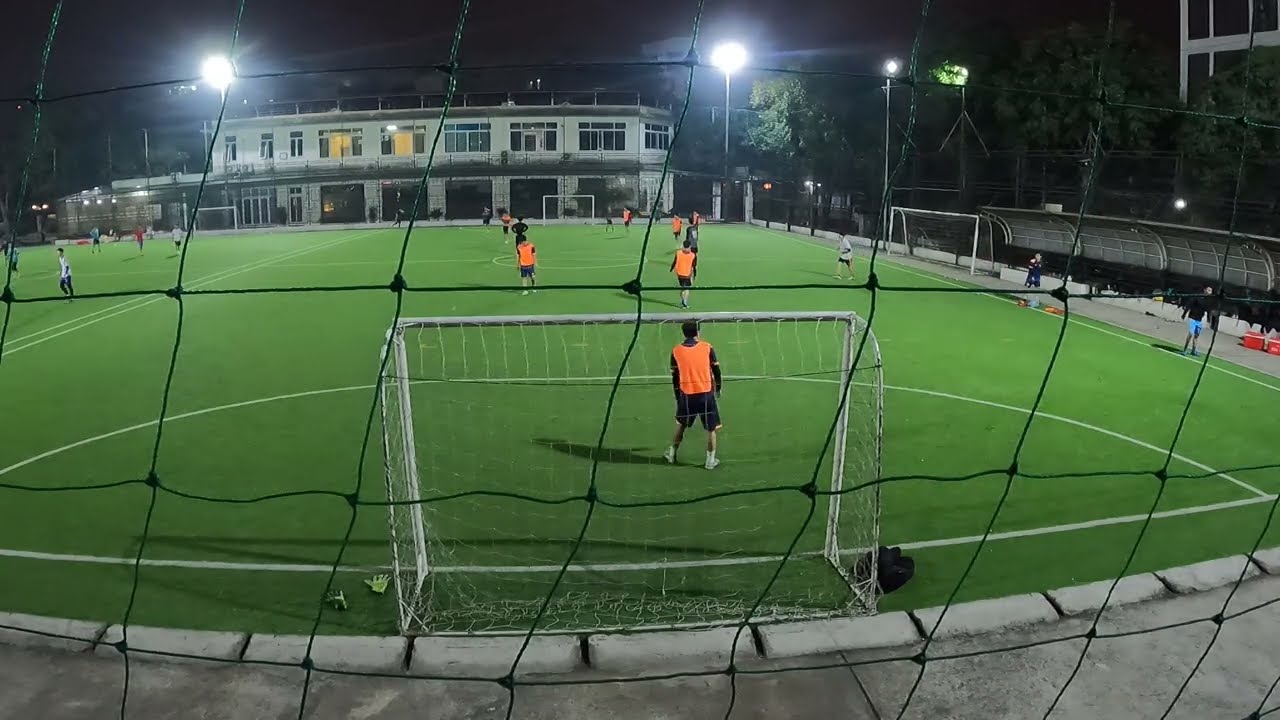This photograph captures a nighttime soccer game on a green AstroTurf field within a city sports complex, visible from behind one of the goal nets. Both teams are actively playing, with one team wearing orange jerseys or pennies. A protective black netting is in front of us, presumably to safeguard spectators. The field is well-illuminated by several overhead floodlights, and there’s another soccer game happening on an adjacent field to the left. In the background, centered slightly to the left, stands a white two-story building, likely associated with the facility, with some of its windows glowing warmly. The sky above is completely dark, emphasizing the nighttime setting.